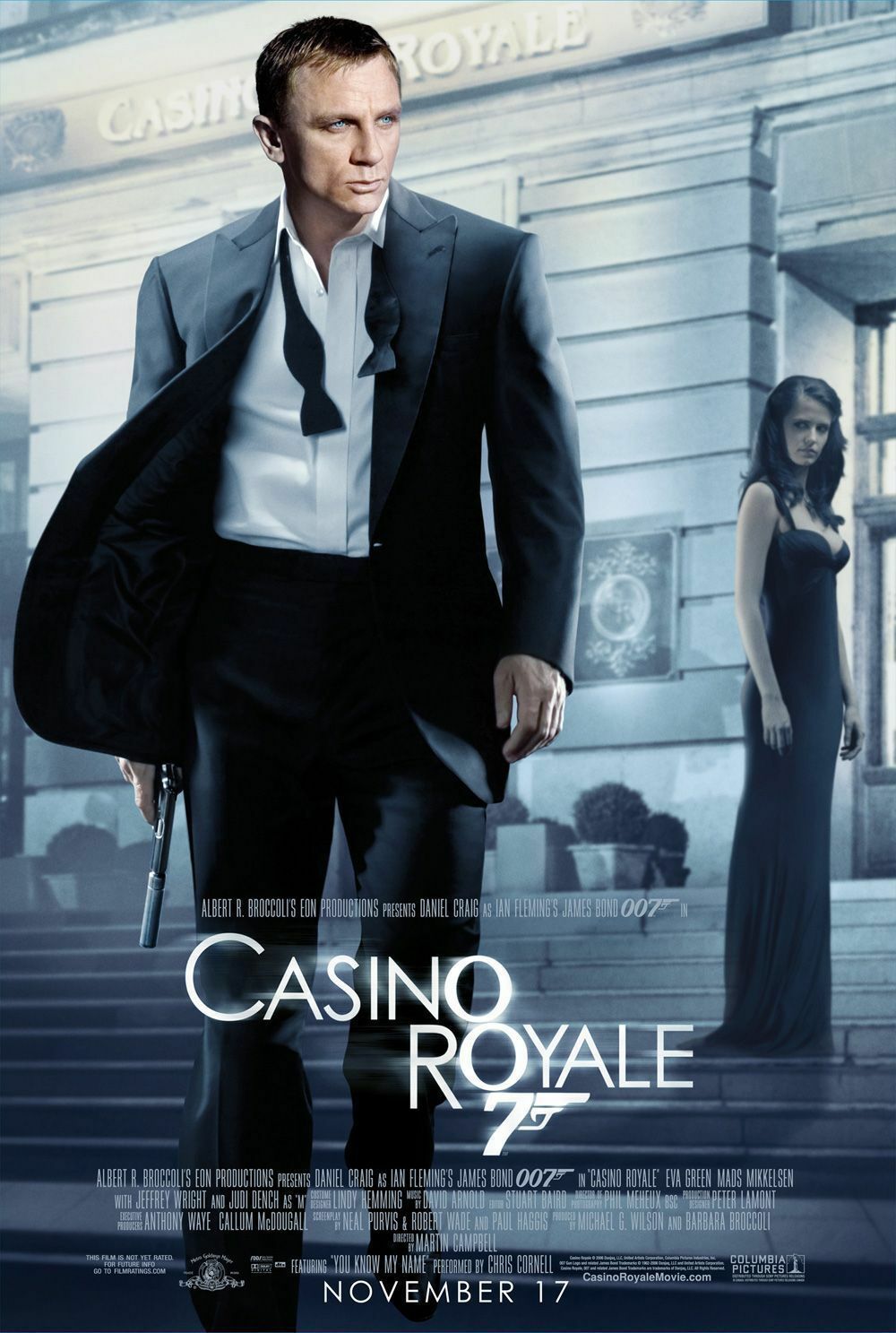The movie poster for Casino Royale showcases a dramatic scene featuring James Bond, portrayed by Daniel Craig, walking toward the viewer on the steps of the Casino Royale. Bond is dressed in a dark blue-to-black suit, with his bow tie undone and his white shirt unbuttoned at the top. His expression is sullen, and he looks down and to the right while holding a silenced pistol at his right side. His short brown hair and blue eyes add intensity to his demeanor. In the background, a woman in a form-fitting black gown, with long black hair cascading past her shoulders, stands about five steps up, observing him. The entire scene is bathed in grayscale tones, adding to the somber mood. Above them, a sign reads "Casino Royale."

The poster’s text prominently displays the movie title "Casino Royale" and the release date "November 17th." Below the title, it reads "Albert R. Broccoli’s Eon Productions presents Daniel Craig as Ian Fleming’s James Bond 007." Additional credits include key cast members Eva Green, Mads Mikkelsen, Jeffrey Wright, and Judi Dench, as well as details about the production team and the crew, such as director Martin Campbell, costume designer Lindy Hemming, and composers. The film is noted to be "Not Yet Rated," with further rating information available at FilmRatings.com. Additional logos, including those of Columbia Pictures and MGM, are displayed alongside the movie's official website, CasinoRoyaleMovie.com.